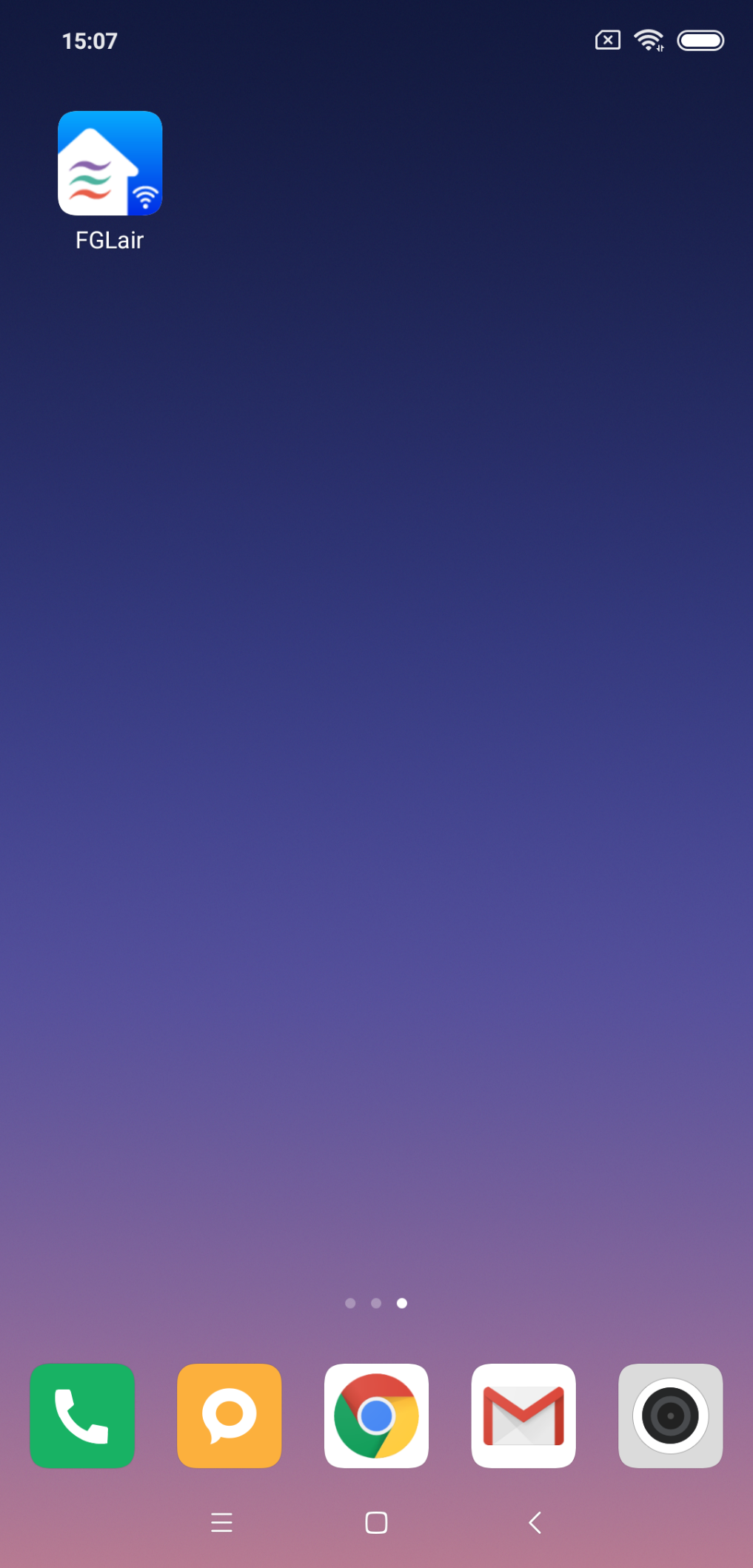This screenshot captures a mobile phone home screen featuring a gradient wallpaper that transitions from light purple at the bottom to deep purple at the top. The time displayed in the top left corner is 15:07 using the 24-hour format. In the top right corner, there are several icons: an "X" icon, a Wi-Fi signal strength indicator, and a fully charged battery icon.

There is only one app icon on the home screen, which belongs to F.G. Lair. This icon features a blue background with a white house silhouette, along with three horizontal approximation lines in purple, green, and red. Additionally, there is a small Wi-Fi icon situated in the bottom right corner of the app icon.

At the bottom of the screen, the typical task bar for the phone is present, containing five icons from left to right: a green phone call icon, a messaging icon on an orange background, a Chrome browser icon, a Gmail icon, and what appears to be a camera or video icon.